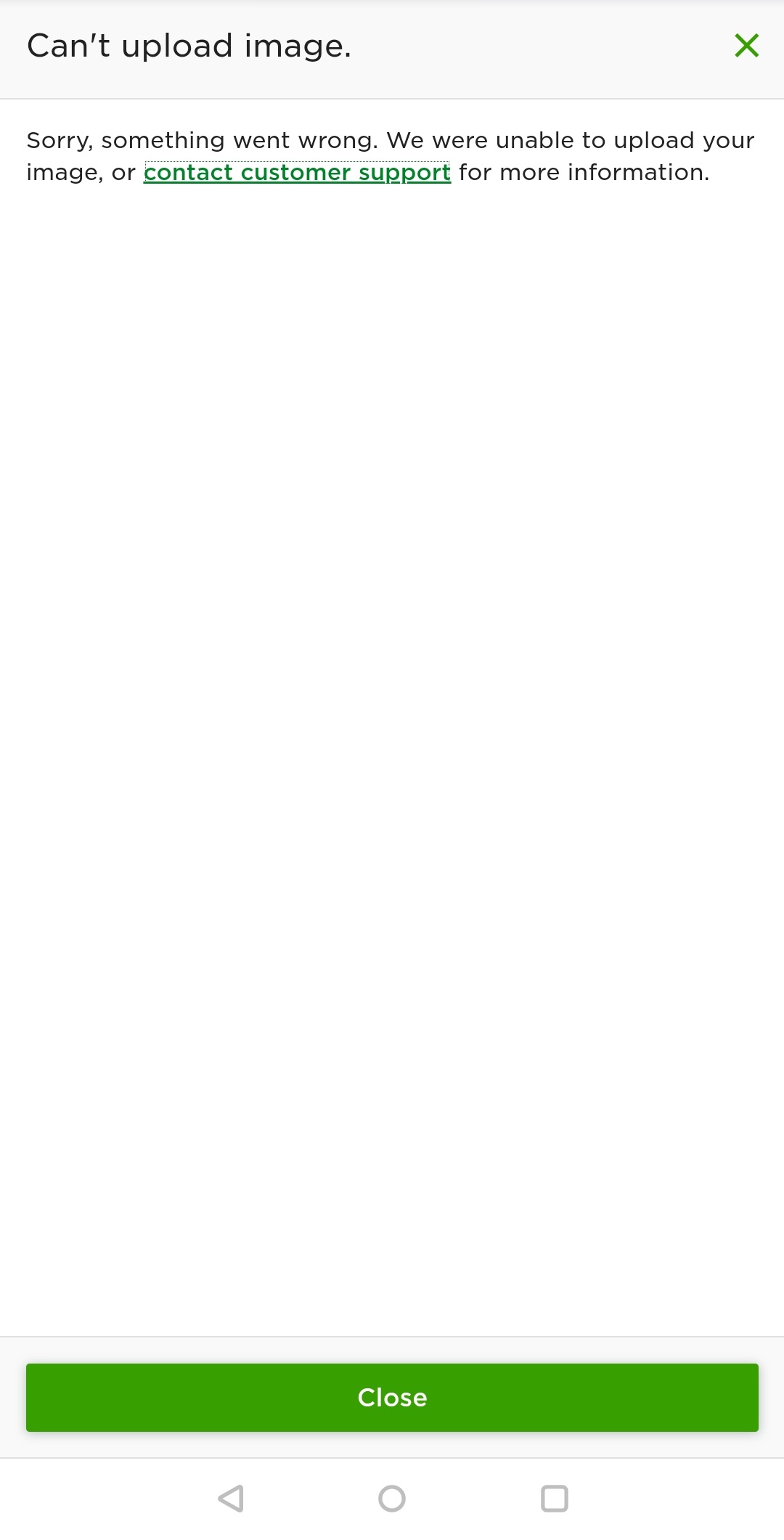A screenshot from an Android app is shown. At the bottom of the image are the Android navigation buttons, including the back arrow, the home button, and the recent apps square icon. The interface is minimalist with a plain white background.

At the top of the screen, within a light gray box, a message reads, "Can't Upload Image." To the right of this message, in green text, is the letter "X." Below this, a notification in smaller text says, "Sorry, something went wrong. We were unable to upload your image. Contact customer support for more information." The phrase "Contact customer support" is clickable and highlighted within a dotted box, indicating a link.

At the very bottom of the screen, a prominent green button labeled "Close" allows the user to exit the message. The overall design of the app interface is simple and uncluttered, focusing on essential information with no additional distracting elements.